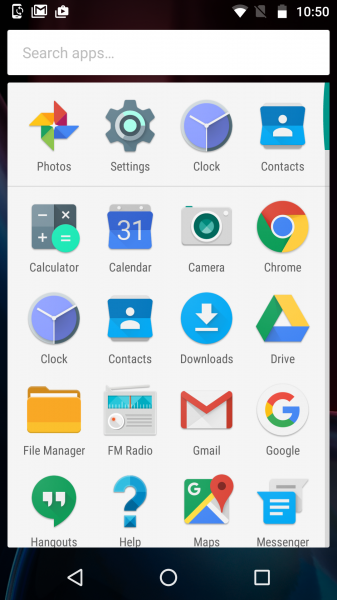This image is a detailed screenshot of a mobile device's home screen, bordered in black. At the top, there's a black header displaying the icons for cell phone signal, Gmail notifications, and the status indicators for Wi-Fi connectivity, battery life, and the current time, which is 10:50. 

Beneath the header lies a white search bar with the prompt "Search apps" in gray text. The main portion of the screen showcases app icons arranged neatly into rows:

- **First Row:** Google Photos, Settings, Clock, and Contacts.
- **Second Row:** Calculator, Calendar, Camera, and Google Chrome.
- **Third Row:** Clock, Contacts, Downloads, and Google Drive.
- **Fourth Row:** File Manager, FM Radio, Gmail, and Google.
- **Fifth Row:** Hangouts, Help, Maps, and Messenger.

A light gray horizontal line separates the first and second rows, adding a subtle division within the app grid.